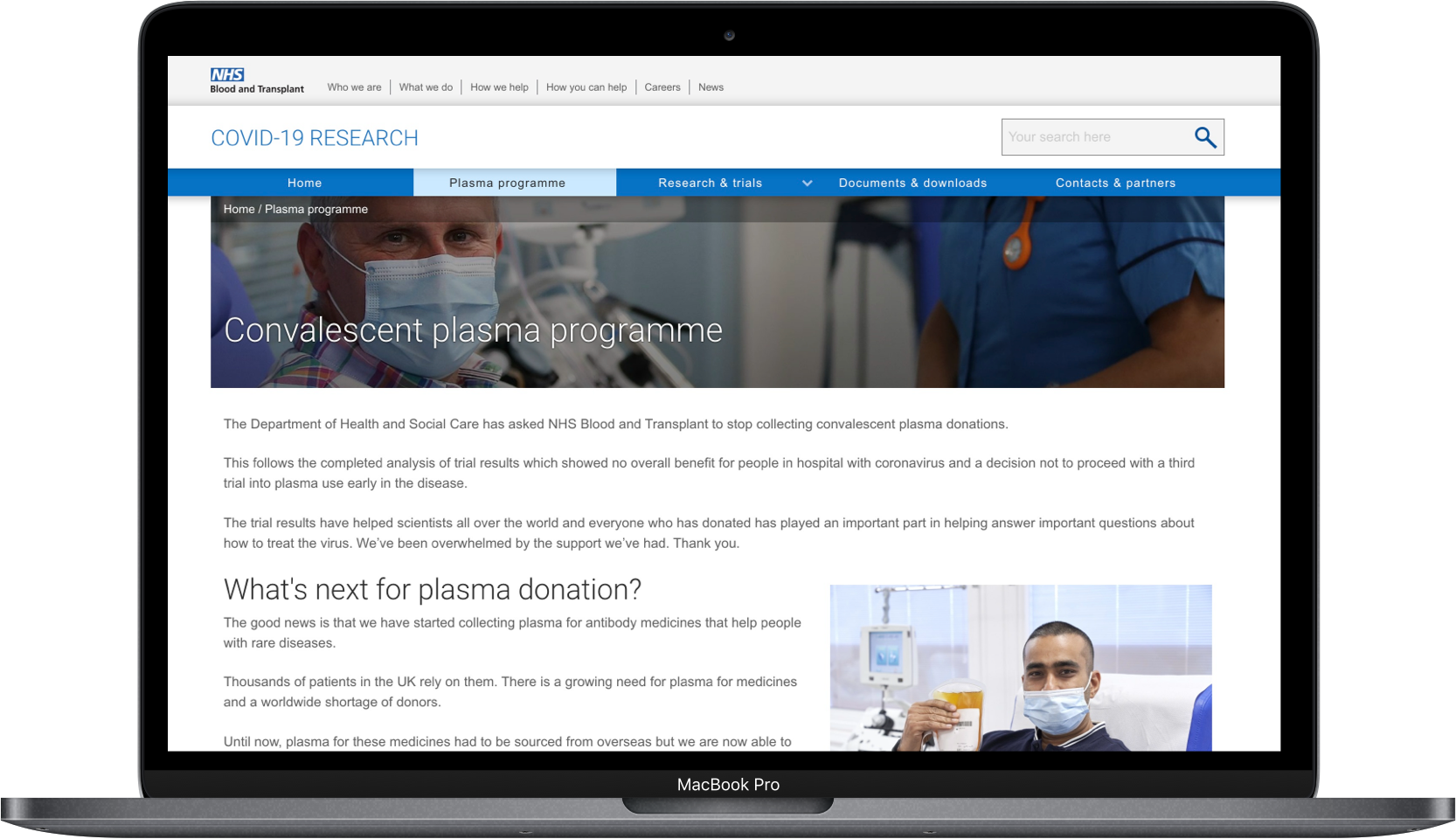This image is a detailed screenshot of the NHS Blood & Transplant website displayed on a MacBook Pro. The website header features the NHS Blood & Transplant logo on the left, followed by a navigation menu with links titled "Who are we," "What do we do," "How can we help," "How we help," "Careers," and "News." On the right side of the header, there is a search bar.

The main content focuses on information about the Department of Health and Social Care's decision to halt the collection of convalescent plasma donations. The text explains that the Department of Health and Social Care has requested NHS Blood & Transplant to stop collecting convalescent plasma donations following a complete analysis of trial results. These results showed no overall benefit for people hospitalized with coronavirus, leading to the decision not to proceed with a third trial into early plasma use for the disease. The information acknowledges the role of donors and the importance of the contribution in answering critical questions about treating the virus, extending a thank you to all who have donated.

The section also introduces the next steps for plasma donation, stating that NHS Blood & Transplant has begun collecting plasma for creating antibodies, which are medicines crucial for treating individuals with rare diseases. It emphasizes the growing need for plasma and the global shortage of donors. Until now, plasma for these treatments had to be sourced from overseas, but the new initiative allows for local collection. The text appears to be cut off at this point.

The screenshot also includes images of a healthcare professional wearing a mask and a patient in a medical setting holding a plasma bag, also wearing a mask, providing a visual context to the information presented on the page.